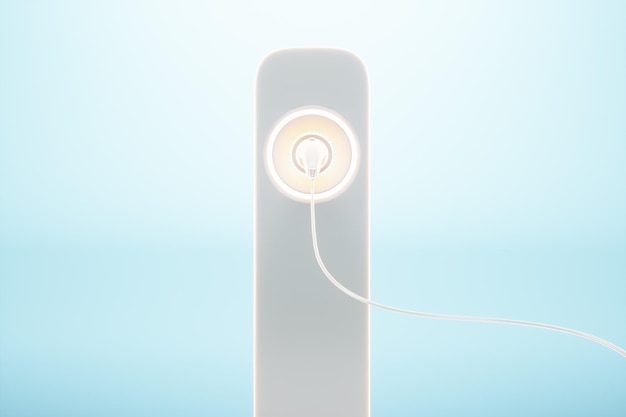In this illustration, we see a highly minimalistic depiction set against a gradient background that transitions from a lighter baby blue at the top to a darker teal towards the bottom. At the center of the image is a slender, rectangular tower resembling a remote control, which occupies about 90% of the vertical space. This tower has straight sides illuminated by a glowing white outline and curves slightly at the top, ending without sharp edges.

Prominently positioned in the upper portion of this tower is a distinctive yellow circle framed by a glowing white perimeter. Emerging from the center of this circle is a white electrical plug or earbud, attached to a cord that curls gently downward and off to the right side, eventually disappearing out of frame. The simplicity of the elements and the clean gradient background lend an airy, almost ethereal quality to the overall composition.